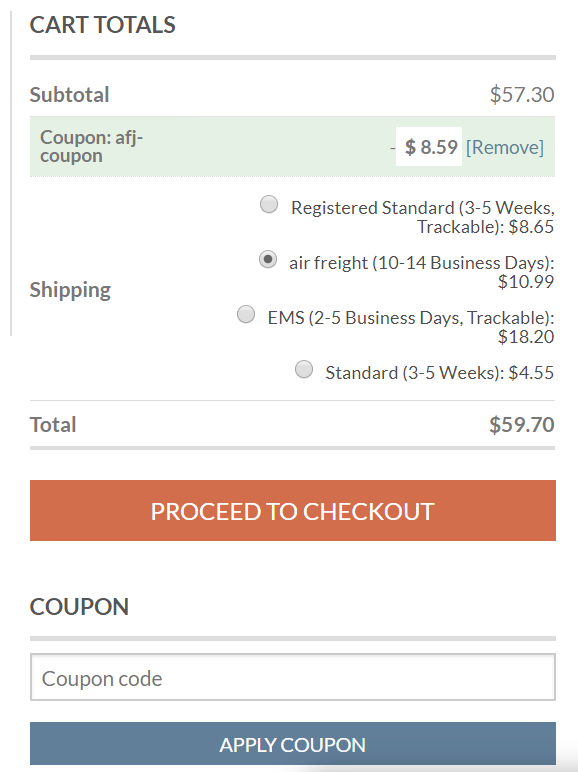A detailed view of an online shopping cart summary is displayed, perhaps from a mobile device. At the top, "Cart Totals" is prominently shown in bold black text. The subtotal for the items is $57.30. A coupon has been successfully applied, reducing the total by $8.59, with the discount highlighted in a bright lime green. Various shipping options are listed: "Registered Standard" (3-5 weeks, trackable) for $8.65, "Air Freight" (currently selected, 10-14 business days) for $10.99, "EMS" (2-5 business days, trackable) for $18.20, and "Standard" (3-5 weeks) for $4.55. The grand total amounts to $59.70. At the bottom, there is a large orange "Proceed to Checkout" button. Additionally, there is a section for entering a coupon code with an "Apply Coupon" button in darkish blue. A "Remove" button in blue text is visible near the applied coupon area. The image is zoomed in closely, offering no further context about the webpage or platform.